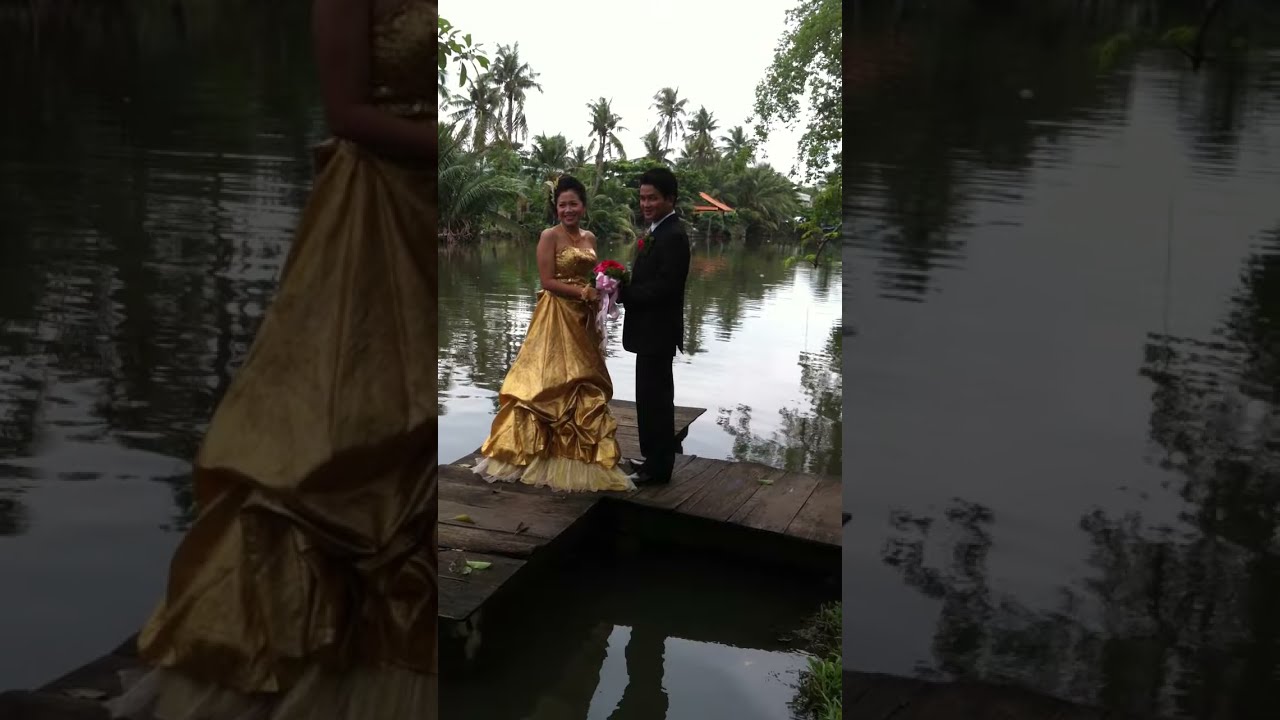This image is divided into three vertical sections. The first and last vertical sections consist of darkened close-ups of the photograph in the middle section. The middle section reveals a serene outdoor setting featuring two young people, who appear to be of Southeast Asian or Polynesian descent, standing on a small wooden platform over a smooth river. Surrounding the river is lush greenery, including palm trees and tropical vegetation, under a light, white sky.

The couple, elegantly dressed as if for a wedding or a formal event, are facing each other. The woman is wearing a floor-length, shiny gold gown with taffeta at the bottom, and her hair is pulled back. She holds a bouquet of pink and red flowers adorned with a pink bow. The man, with short black hair, is dressed in a black tuxedo with a red boutonniere on his lapel, possibly also holding the bouquet. The scene exudes a festive and romantic atmosphere, typical of settings found in Vietnam, Thailand, or other parts of Southeast Asia.